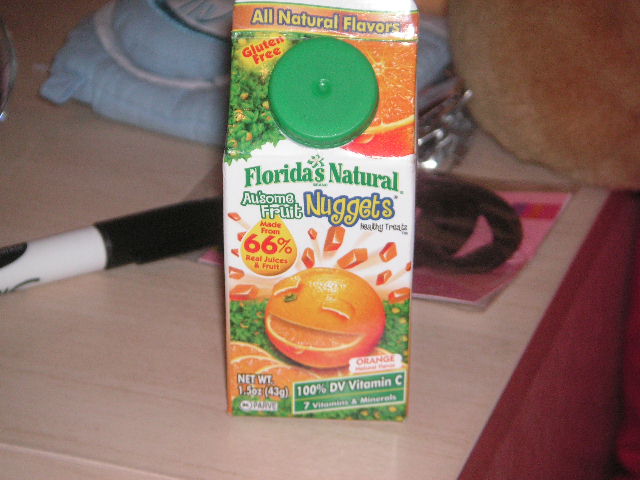The image is a color photograph capturing a 1.5-ounce container of Florida's Natural Awesome Fruit Nuggets prominently placed in the center. The container boasts vibrant hues of green, orange, and yellow, and is adorned with a large, proportionally-sized green cap. This single-serving pack of fruit nuggets is made from 66% real juices and fruits, offering all-natural flavors and gluten-free ingredients. It claims to provide 100% of the daily value (DV) of vitamin C along with seven essential vitamins and minerals.

The container features a playful cartoon orange with one eye winking and a slice cut out from its body, from which small orange cubes or pieces seem to float out. There's an orange stripe at the top that reads "All Natural Flavors" in yellow, while a background of orange orchards and a white expanse dotted with tiny orange bits enhances the overall design. The product description prominently includes the phrases "Florida's Natural" and "Awesome Fruit Nuggets" in green and white text respectively.

The scene is set against a light brown wooden countertop, with a Sharpie marker and a lanyard visible nearby, adding a casual touch to the setup. Blurred in the background are hints of pillows or blankets in brown and blue hues, giving context to the everyday environment of the photograph.